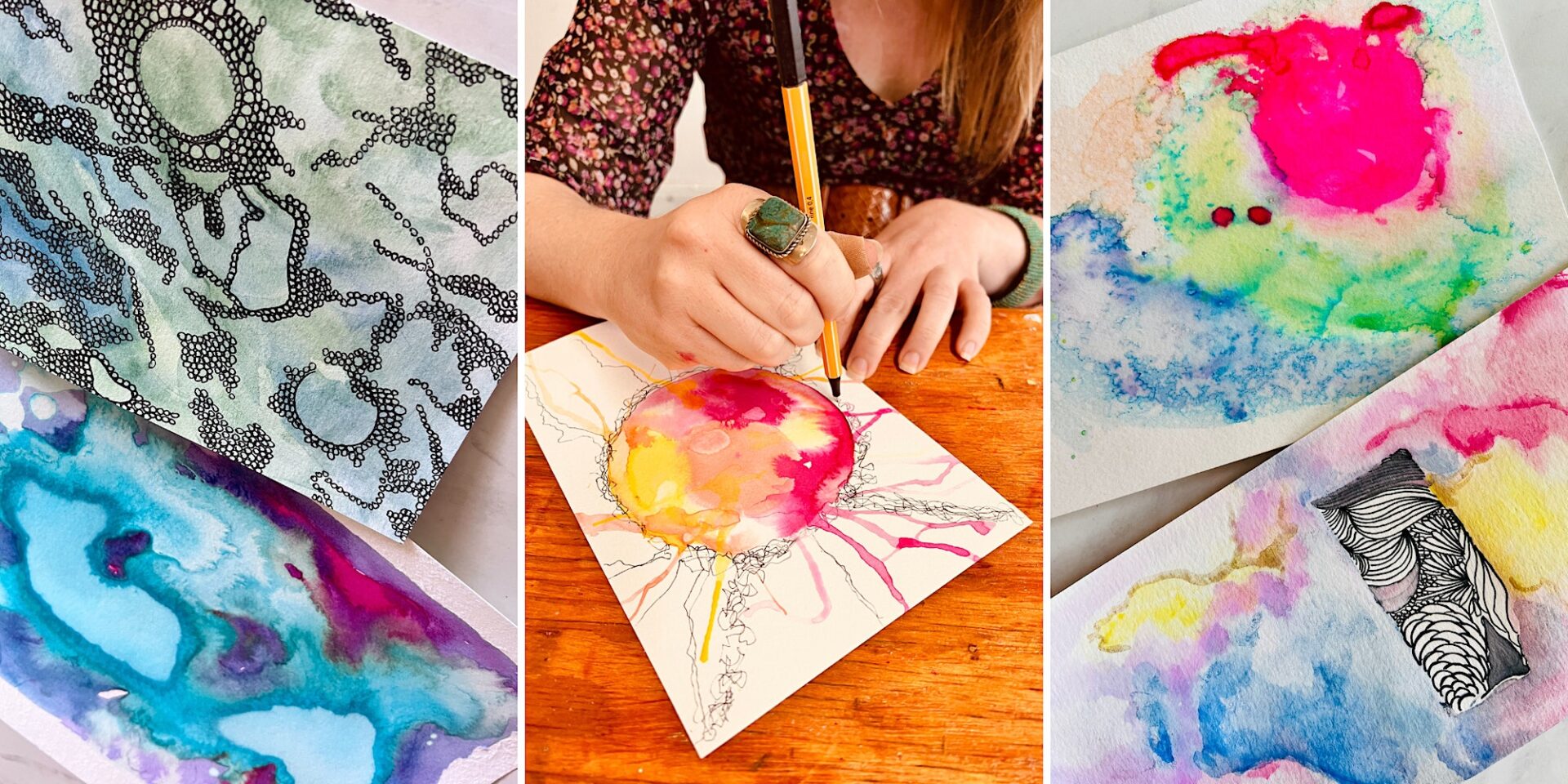The image features a three-panel composition. On the left side, there are two small canvases laid down, each showcasing unique artwork. The bottom canvas presents a vibrant mix of blue, purple, and red hues, resembling a tie-dye pattern. The top canvas displays a bluish background adorned with intricate black designs, featuring multiple small circles forming various shapes.

In the center panel, a woman with auburn hair is depicted in the process of creating an illustration. She is seen from a slight angle, revealing a bit of her hair and the floral-patterned shirt she's wearing, which has long sleeves possibly rolled up. A distinctive green ring adorns her pointing finger as she holds a yellow and black drawing utensil. She is drawing on a piece of white paper that has a central circle with lines radiating from it, surrounded by yellow, pink, and red colors. This paper rests on a brown wooden tabletop.

The right panel contains two more artworks on canvas or paper. Both pieces exhibit a splotchy, watercolor style with random colors such as red, green, and blue. The bottom artwork also includes a black and white illustration, which resembles an arrangement of plants or feathers forming a blocky shape. The composite image collectively highlights the artist's ongoing work and past creations, emphasizing the dynamic and colorful nature of her artistic process.